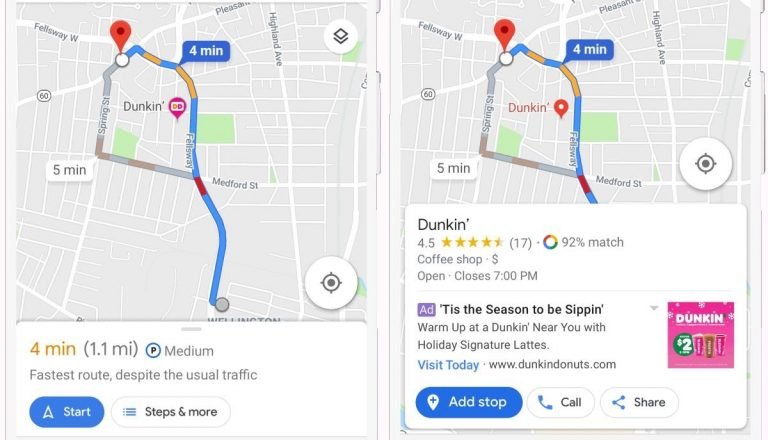A map displays the fastest route to Duncan, which is a 1.1-mile journey expected to take approximately four minutes despite the usual traffic. The route, ideal for those who wish to reach their destination quickly, highlights key steps and stops along the way. The destination, Duncan, enjoys a high rating of 4.5 stars, making it a popular spot during the festive season for enjoying a warm beverage.